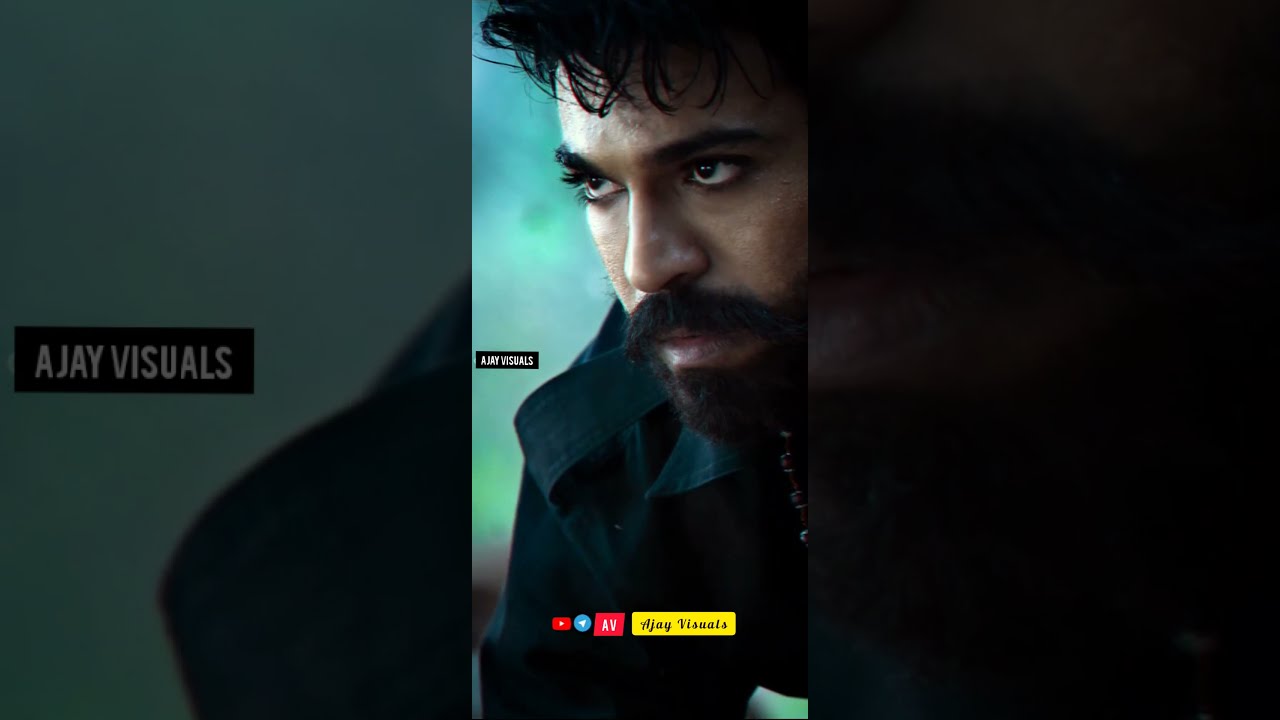This cell phone photo features a digital image of a South Asian or Middle Eastern man with white skin, dark black hair, and a distinctive black mustache that connects to a well-trimmed beard. He has an intense and serious expression on his face, gazing towards the left of the frame. The man is dressed in a black jacket with epaulets and a beaded necklace around his neck, adding a rugged yet composed appearance.

The photograph itself seems to be displayed with some digital framing, creating fragments of the image on either side, which are larger but less clear versions of the central picture. The background is a mix of turquoise, blue, and green hues.

To the man’s left, there is a black rectangle with white text that reads "AJAY visuals," also repeated in a yellow rectangle at the bottom of the image along with several social media buttons. These include a red play button for YouTube, a blue circle logo, and a red AV button, making the image look like a promotional or digital content piece.